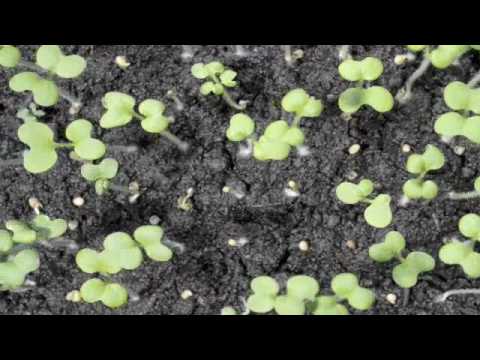This image provides a detailed, overhead view of a garden scene featuring freshly sprouted seedlings emerging from dark, moist soil. The soil, almost black due to its wetness, is dotted with small white specks of perlite. The seedlings, some still adorned with seed shells, are scattered across the ground, their light green, kidney-shaped leaves appearing in pairs around slender, green stems. These tiny plants, standing roughly one to two inches tall, protrude towards the camera, contrasting vividly with the brown and black soil. The overall setting is zoomed in closely on the earth, capturing the fragile beginnings of new growth as they break through the surface. The image is rectangular with black and white letterboxing at the top and bottom, with no additional text or significant features.